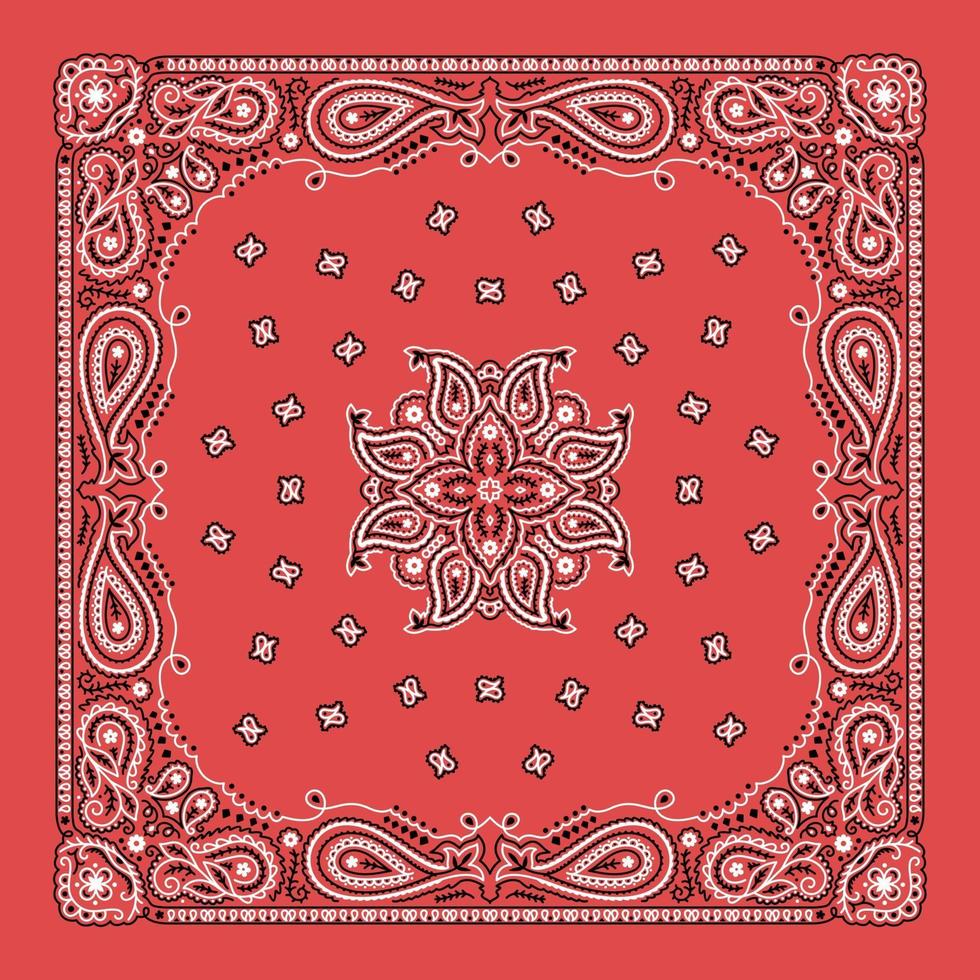The image depicts a detailed illustration of a red bandana design, reminiscent of those traditionally worn by cowboys. This square piece features a rich, solid red border on the outside. Within this perimeter, the design intricately incorporates a paisley pattern, abundant with teardrop and leaf shapes. Notably, there is a white scroll-like line adorned with black diamond shapes and dots that loops around the inside of the red border. The central area of the bandana continues the red background, interspersed with small black and white symbols. Prominently, a star-like flower arrangement occupies the middle, surrounded by round dots. This central motif is surrounded by paisley shapes on all four sides, creating an ornate, symmetrical design. Each corner of the bandana also features a small flower-like detail, emphasizing the folk art aesthetic. The elaborate pattern suggests it could either be a wearable bandana or a piece of decorative folk artwork.